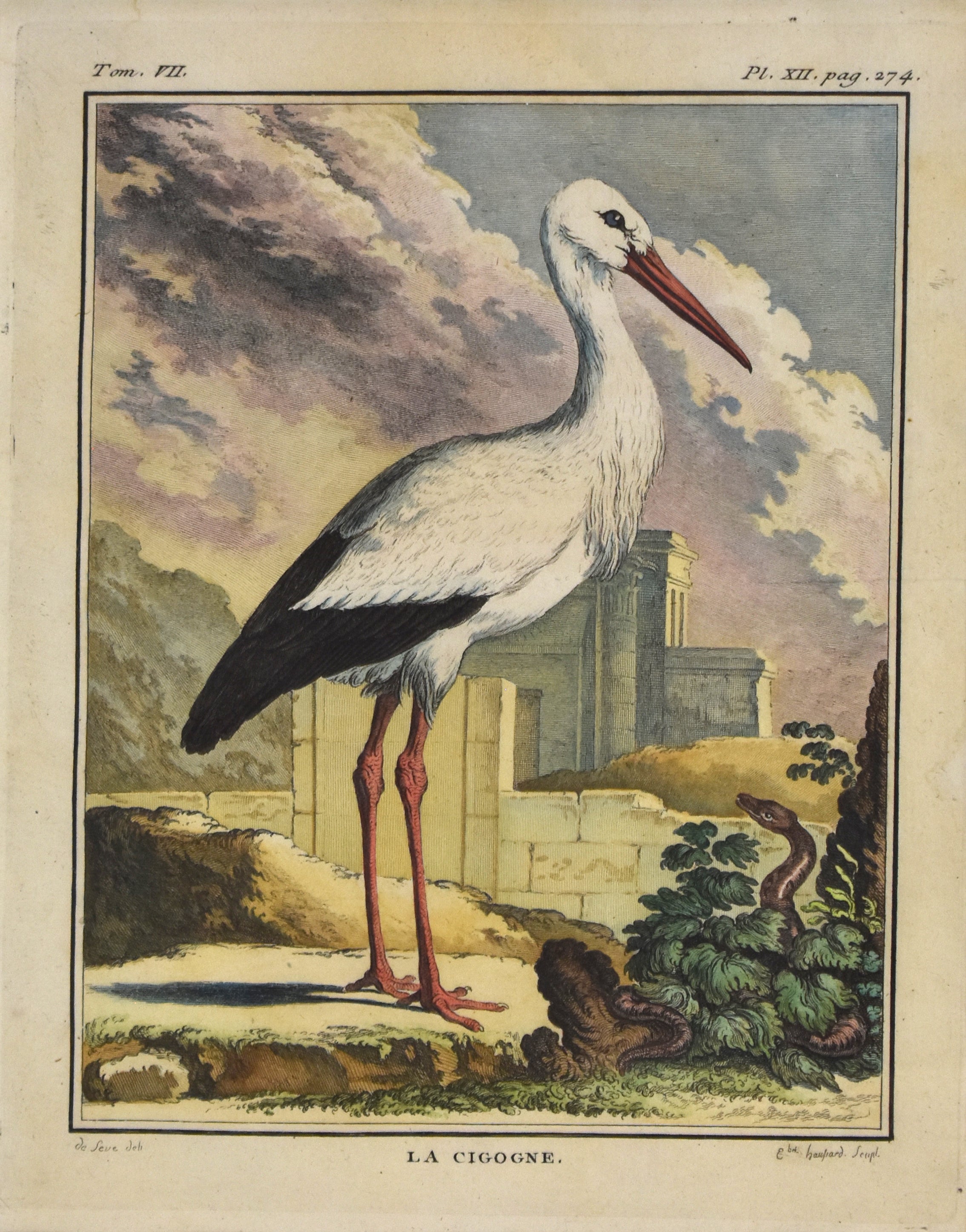This is an antique illustration with a cream-beige, aged paper background, bordered by a thin black line. At the top left, the text reads "Tom VII," while the top right has "Page 274." The bottom features the title in bold, "LA CIGOGNE." The image portrays a large bird, likely a pelican or heron, with a white body, black-tipped back feathers, long orange legs, and a striking orange beak. It stands in a detailed outdoor scene with crumbling stone buildings similar to a coliseum, green hills to the left, and various rock formations. The background features a sky filled with light purple and yellow hues, accompanied by white clouds. At ground level, there are bushes and two brown snakes; one curls around a plant on the lower right, its head raised towards the bird.